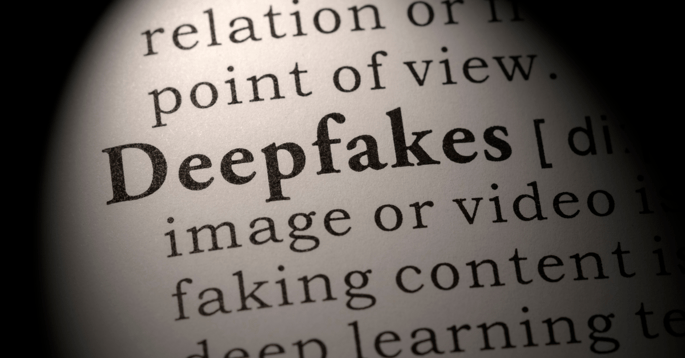This image features a close-up of text, possibly from a book or document, with a distinct focus on the bolded phrase "deep fakes" prominently placed in the center. The text is black against off-white, somewhat beige background, which is partially shadowed, particularly around the edges, giving it a vignette effect. Surrounding "deep fakes," you can also make out fragmented phrases like "relation of," "point of view," "image or video," "faking content," and "deep learning," though these are cut off and partially obscured. The light source seems to shine from the top left, accentuating the central bold text while the edges fade into shadows, making it difficult to read the entire context. The focus on the term "deep fakes" suggests its significance, with all other words appearing secondary and less distinct.